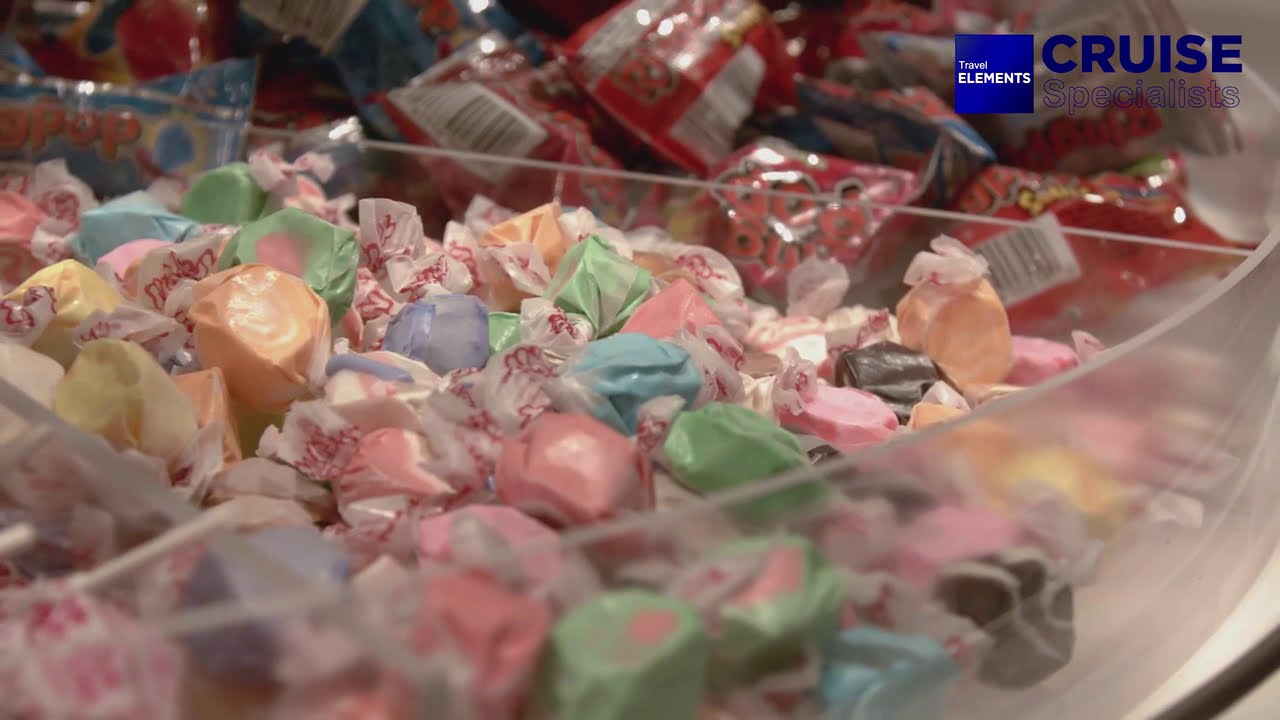This horizontal rectangular close-up image depicts a colorful assortment of water taffy candies, all wrapped in almost clear cellophane wrappers, arranged within sections of a transparent, round plastic tray. The foreground section is vibrant with various colors including green with pink centers, solid yellows, solid pinks, brown with stripes, solid oranges, orange with white stripes, and blues. Each compartment is separated by clear plastic barriers. In the compartment above and to the left, there are red and white bags that seem to say "POP ROCK," though this area is somewhat blurry and partially obscured. The upper left corner shows another compartment barely visible, containing blue packaging with the word "POP" on it. Across the top of the image, the words "CRUISE SPECIALIST" are prominently displayed in bright blue and white all-caps lettering, alongside a blue square with white letters spelling "TRAVEL ELEMENTS." The entire setup appears to be placed on a beige surface, making for a visually enticing and organized display of treats.